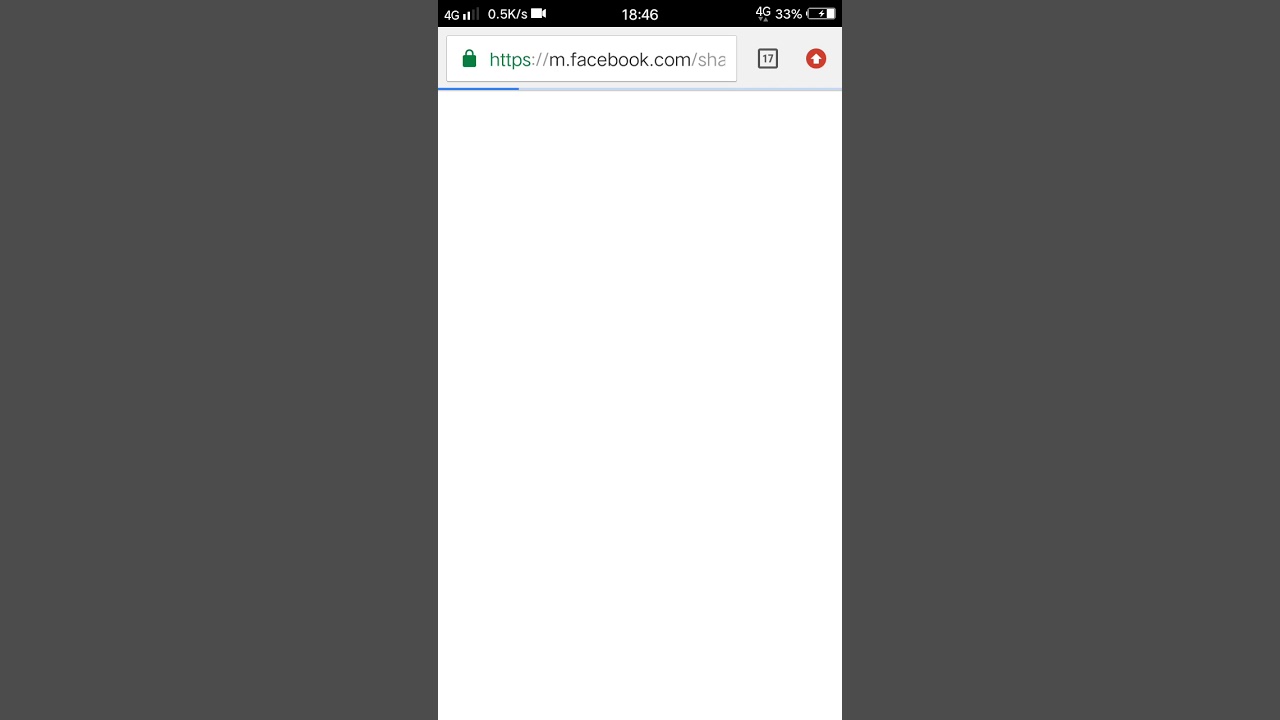A smartphone screen displays a loading Facebook page. The status bar at the top of the screen shows a 4G connection with 2 out of 4 signal bars, a data rate of 0.5 Kb/s, and a battery level at 32%. The time indicated by the phone is 18:46. The screen is predominantly white with green accents, featuring an HTTPS URL for the mobile version of Facebook at the top. A gray square, labelled 17, and a red arrow pointing upwards are visible on the loading screen. These elements are centrally aligned, indicating that the loading process is still ongoing.